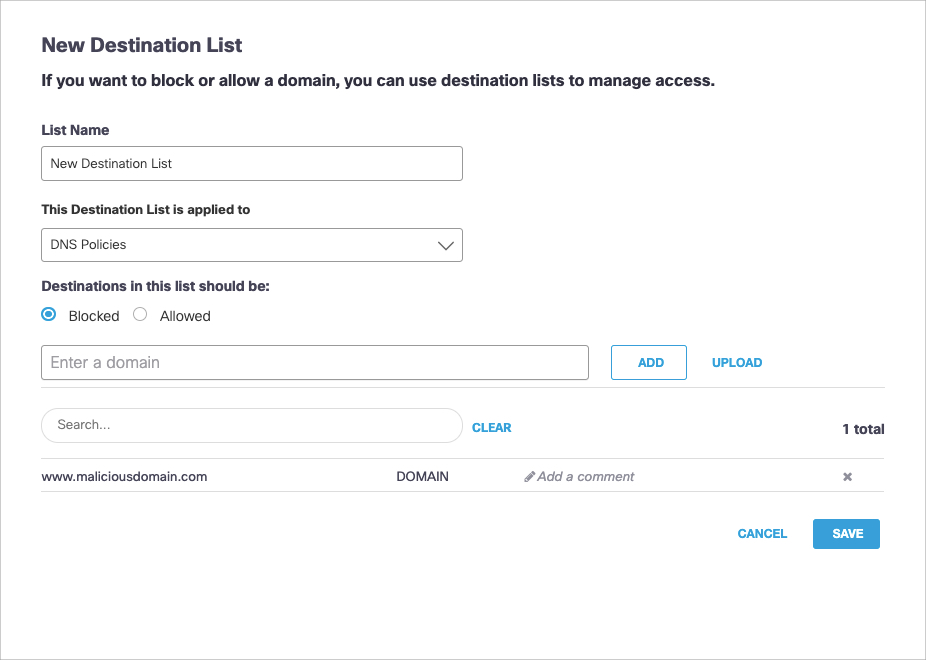A cropped screenshot exhibits an enlarged white interface box. At the top-left corner, in bold black letters, the title "New Destination List" is prominently displayed. Directly below, a description reads: "If you want to block or allow a domain, you can use the destination list to manage access."

Under this text, the label "List Name" is positioned to the left, with an accompanying text bar below it. Within this bar, the phrase "New Destination List" is typed. Moving down, the text "This destination list is applied to" is followed by a dropdown menu set to "DNS Policies."

Further below, the instruction "Destinations in this list should be" is adjacent to radio buttons labeled "Blocked" and "Allowed," with "Blocked" selected. Next, a long text entry box contains the prompt "Enter a domain," accompanied by "Add" and "Upload" buttons to its right.

Towards the bottom-left, a search bar showing the word "Search" in grey is positioned beside a blue "Clear" button. Below, a text box displays the URL "maliciousdomain.com" with "Domain" in capital black letters to its right. Adjacent to this is another text box labeled "Add a comment" with an "X" button to its right.

Finally, at the bottom-right corner, there are buttons for "Cancel" and "Save," with the "Save" button highlighted in a blue box.